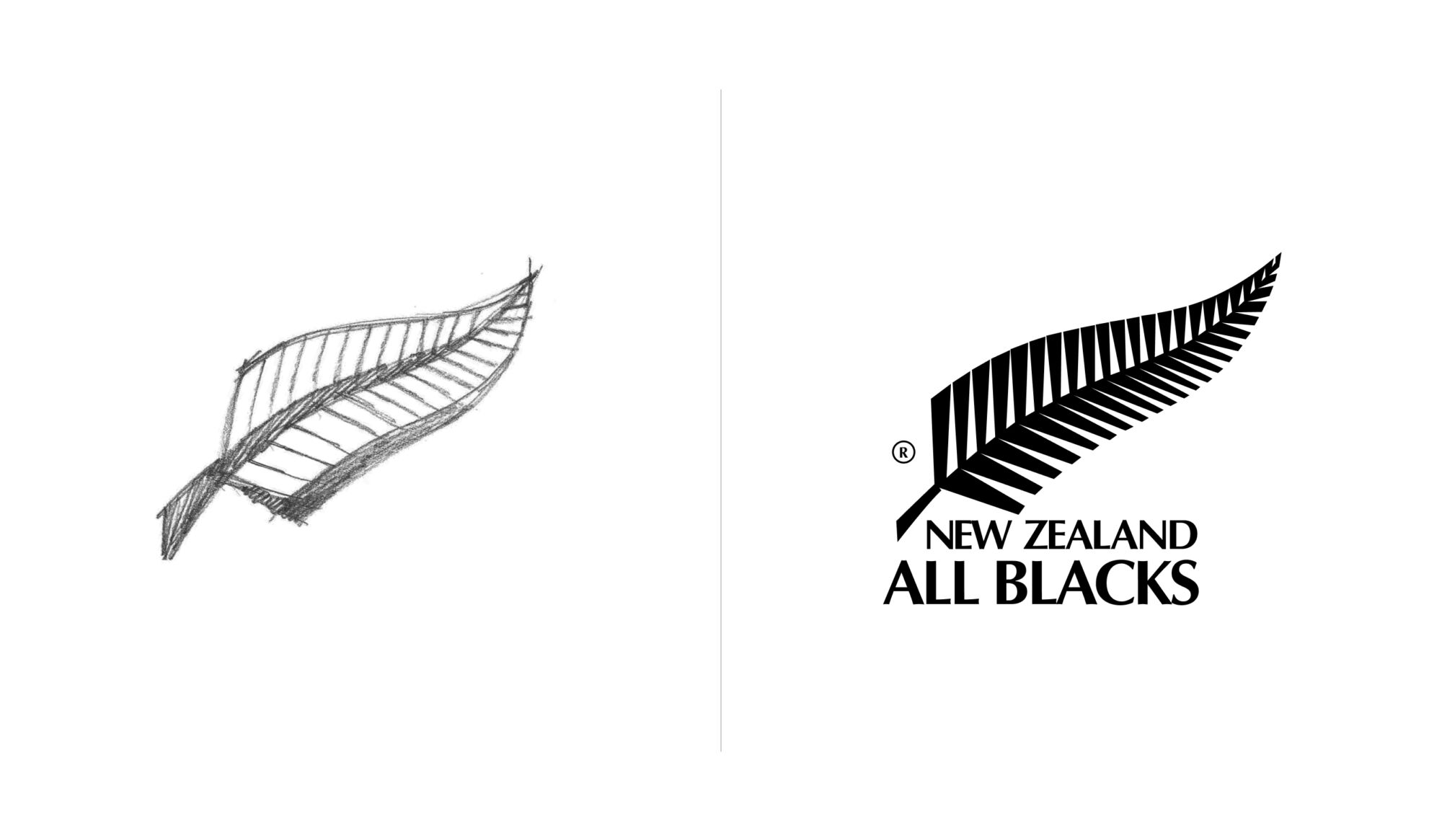The image illustrates the evolution of a logo design, split into two panels. The left panel features an initial pencil sketch of a black feather or fern leaf, rendered in shades of gray on a white or slightly off-white background. This sketch appears hand-drawn, characterized by intricate lines extending from a central vein, culminating in a stem-like base. The right panel presents the finalized logo, a polished black vector graphic of the feather or fern leaf, now accompanied by a registered trademark symbol. Below this refined image, the text "New Zealand All Blacks" is inscribed in a bold, sans-serif font, harmonizing with the sleek, modern design of the logo. A thin black line separates the two panels, clearly demarcating the transition from conceptual sketch to completed design.